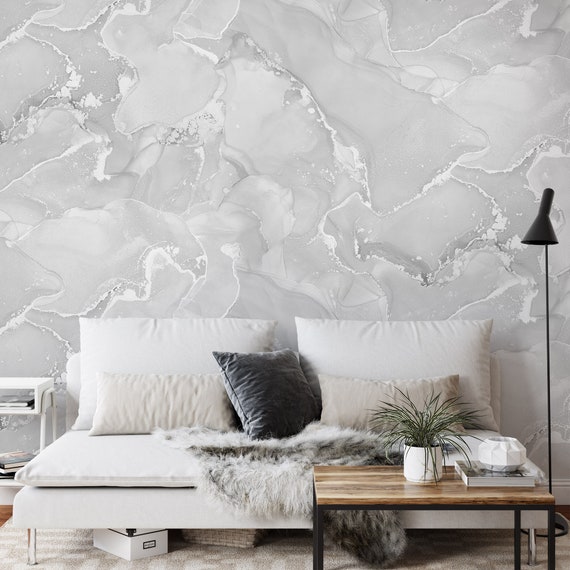The image features a modern and cozy living room with a stylish daybed or couch set against a distinctive gray and white wall that has a marbleized, watercolor effect resembling granite. The daybed is adorned with multiple pillows, including two white ones leaning against the wall, a dark gray velvet pillow in the center, and a tan pillow. Draped across the middle of the daybed is a luxurious fluffy white faux fur throw. 

In front of the daybed, there is a sleek coffee table characterized by a light-colored wooden top with mixed shades of white, light, and dark brown, supported by metal legs. Atop the table sits a white plastic planter containing a vibrant green plant with grass-like leaves. Additionally, a book and a vase are placed on the table. To the right of the daybed stands a modern black floor lamp with a long rod and a lamp at the top, adding to the room's contemporary ambiance.

Beneath the daybed, there is a visible white storage box on the bottom left side. The floor features a tan and white rug that complements the hardwood pine floor. The overall setting is stylish yet welcoming, combining both aesthetic appeal and functional design.